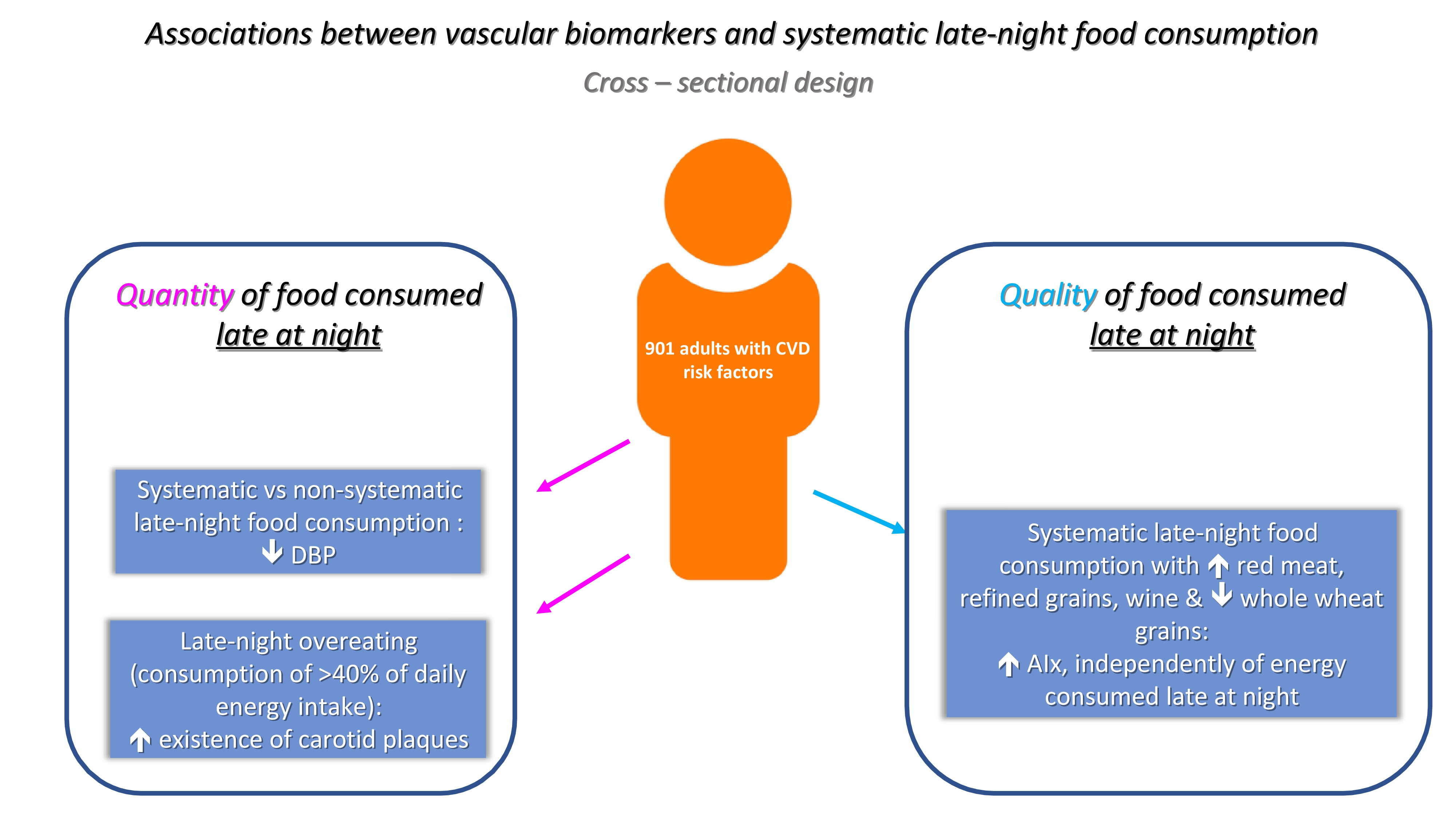The image is an educational poster, likely intended for a school setting, focusing on the associations between vascular biomarkers and late-night food consumption using a cross-sectional design. Dominating the center is an orange human silhouette labeled "901 adults with CVD risk factors." Above this figure, the title reads, "Associations between Vascular Biomarkers and Systematic Late-Night Food Consumption," with "cross-sectional design" written underneath. To the left of the silhouette, a box outlined in purple contains the text "Quality" in purple, followed by "of food consumed" in black and "late at night" underlined. To the right, a blue box contains "Quantity" of food consumed late at night. Purple arrows from the silhouette point to the box on the left, while a blue arrow points to the box on the right, visually linking the central figure to both descriptions.